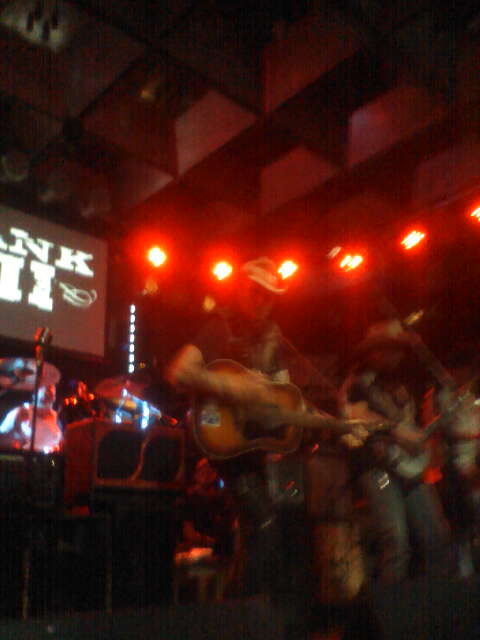This is an indoor photo of a band performing on a stage, captured from an audience perspective. The image is quite blurry, making it challenging to discern all the details. The ceiling of the tall building is adorned with multiple red stage lights, creating a glowing ambiance that might contribute to the blur. In the foreground, two men are visible, each wearing cowboy hats, black t-shirts, and jeans. Both are playing guitars pointed towards the right of the picture. A silver microphone stand is positioned in the bottom left. In the background, there's a drum set and potentially another band member, possibly playing a keyboard or another instrument, though his details are unclear. A large screen is present behind the band, displaying letters in white over a black background, showing an "N" and "K" on the top line, with an "I" on the bottom, obscured and incomplete.